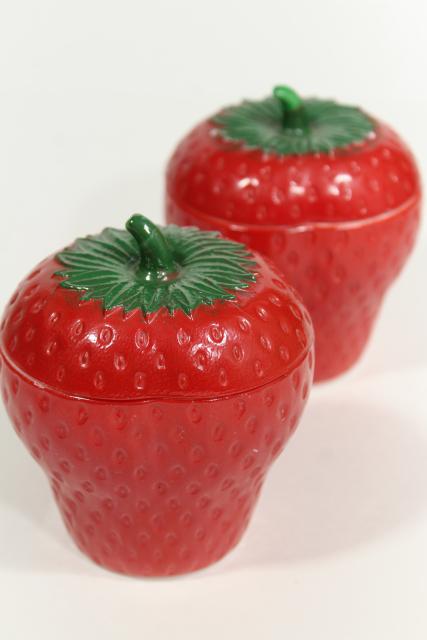This photograph features two lifelike, strawberry-shaped containers set against a white background. Both jars are an intense, deep red with glossy, reflective finishes that showcase detailed depressions where strawberry seeds would typically be. Each container is topped with a green stem-like lid that appears to be removable, possibly with an insert mechanism. The jars are identical and have flat bottoms, allowing them to stand upright. While the container in the back is slightly blurred, the one in the front is prominently displayed, highlighting its vivid color and intricate design. These jars may be made of glass or ceramic, as suggested by their shiny, smooth surfaces and the semi-opaque nature of the green lid, visible in the background jar.